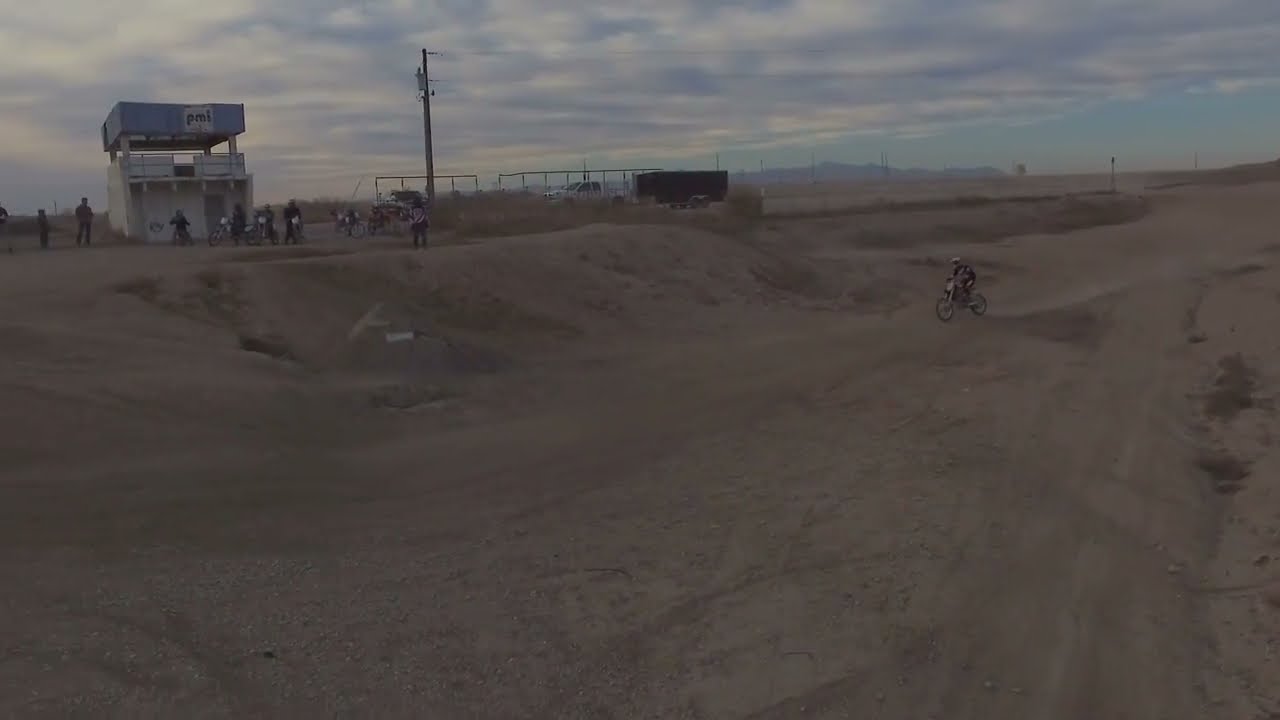The photograph captures a dusty motocross track under a light blue, clouded sky, suggesting late afternoon or early evening with minimal sunlight. The mostly dirt and sand track is set in an ATV park, characterized by worn paths and sporadic vegetation along hilly areas. A central white structure topped with a blue awning stands towards the top left, reminiscent of a concession stand, and is surrounded by spectators and their stationary motorcycles. In the distance to the right, a rider with a white helmet can be seen in action on the track. Nearby, a truck and a large toy trailer are parked within a fenced area. Telephone poles and wires crisscross the image, and faint mountains can be discerned in the background, adding to the rugged outdoor setting.